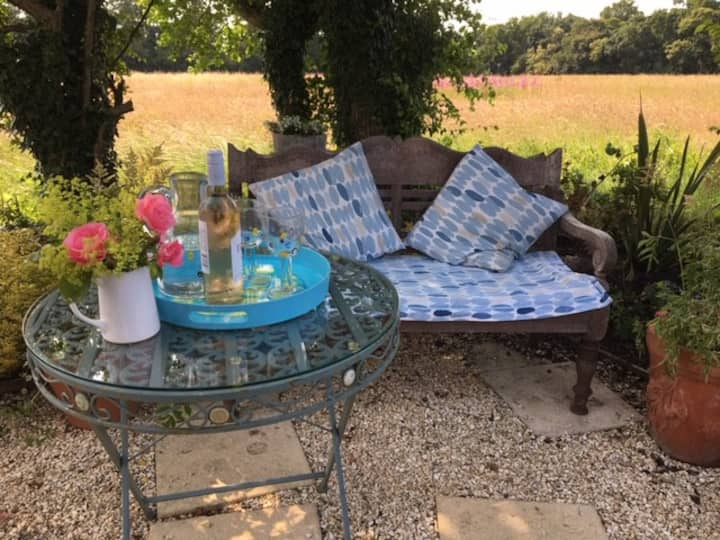This image captures a serene backyard patio scene bathed in gentle daylight. In the foreground, a sage green, foldable metal table with a glass top hosts a blue tray containing an unopened bottle of rosé, two wine glasses, and a carafe of water. Adorning the table is a white enamel watering can filled with freshly picked pink roses and green grasses. Gravel and stepping stones form the ground surface, creating a rustic charm.

Adjacent to the table is a wrought iron bench or loveseat, featuring a blue cushion with two patterned pillows adorned with blue ovals and beige accents. Behind the bench, a rustic planter in rust color holds vibrant green plants and additional pink flowers. This outdoor seating area is framed by lush greenery and potted plants, leading the eye towards a peaceful expanse of farmer's fields with a touch of tan and golden hues.

In the distance, a dense line of trees borders the fields, merging with the clear sky, further enhancing the tranquil rural ambiance of this well-maintained and inviting patio space.